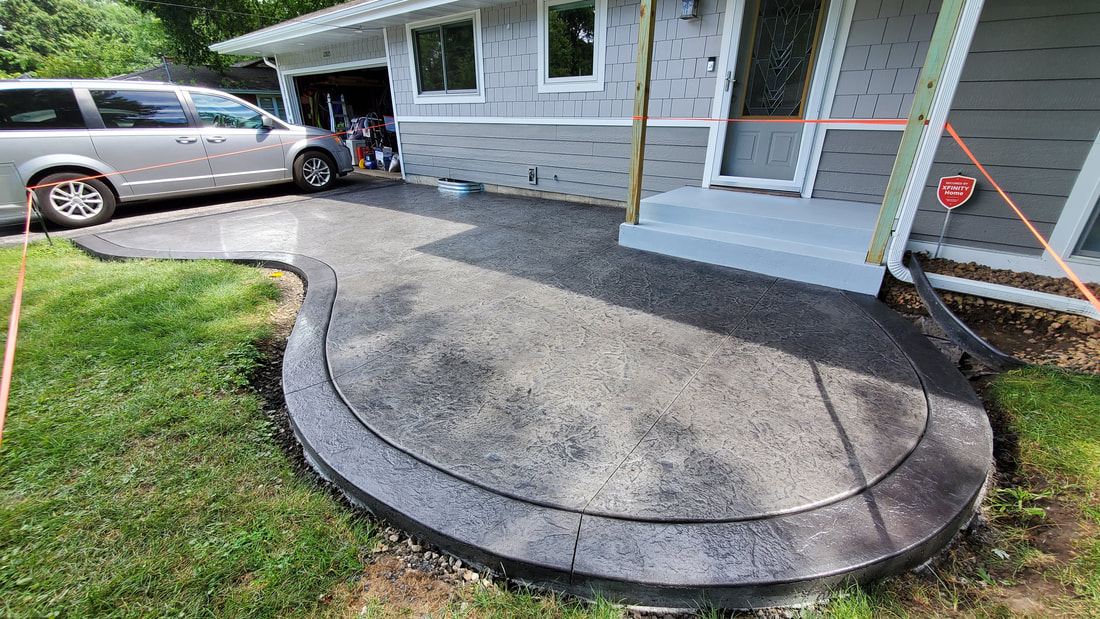This full-color photograph, taken outdoors on a sunny day, showcases a beautifully remodeled front walkway of a gray house with cedar shake siding. The square image captures multiple elements of the aesthetically pleasing entrance. The new walkway, made of high-quality concrete, features a unique, curving design that is reminiscent of a goldfish shape and extends gracefully from the driveway to the front door area, which includes white steps. A gray minivan is parked to the left, in front of the garage, and red tape cordons off the area, indicating the recent completion of the construction. The scene is framed by vibrant green grass and a few trees visible in the upper left-hand corner, with large windows adding to the architectural charm of the home.